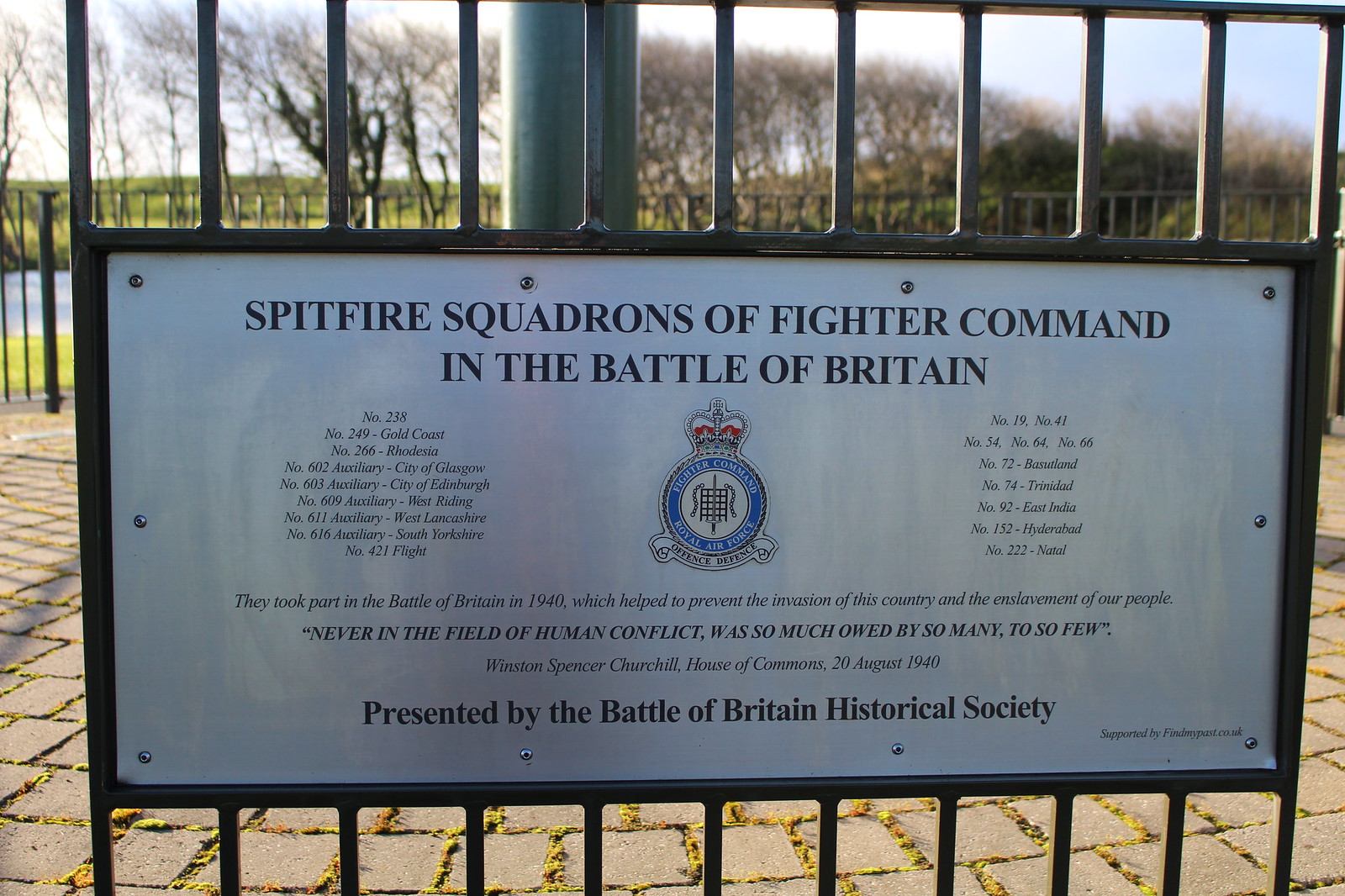The photograph features a detailed informational placard embedded within a black wrought iron fence. The rectangular placard, fabricated from a white stainless steel-like material, is securely mounted with flat-head screws—two on the top and bottom edges, and one on each side, plus additional screws in the corners for extra stability.

The text of the placard highlights the "Spitfire Squadrons of Fighter Command in the Battle of Britain," listing units such as number 238, number 249 Gold Coast, number 266 Rhodesia, number 602 Auxiliary City of Glasgow, number 603 Auxiliary City of Edinburgh, and number 609 Auxiliary... It is inscribed with a dedication mentioning that these squadrons played a crucial role in the 1940 Battle of Britain, a pivotal defense that prevented the invasion of the country and its people. The text further includes a famous quote about the heroics of these squadrons and notes that the placard is presented by the Battle of Britain Historical Society.

Positioned centrally within the fence, the placard also features a crest that draws the viewer’s attention. The background of the image shows another fence, a grassy area, a body of water, and several leafless trees, adding depth and context to the setting.